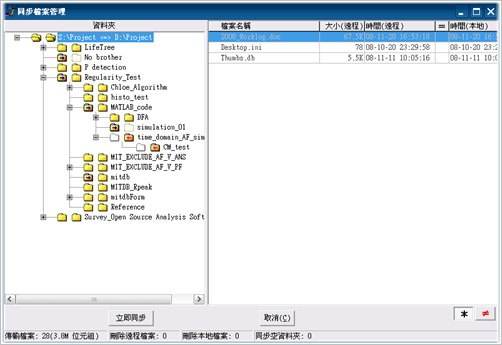The image is a screenshot of a computer screen displaying a browser interface in Chinese, likely Mandarin. The screen is divided into two panels. The left panel features a folder tree with both expanded and collapsed folders. The primary folder is named "project," containing subfolders with names such as "live tree," "no brother," "P detection," "regularity test," "Cole algorithm," "histo test," "math lab code," "FDA simulation," and "a one-time domain AF," among others. The icons next to the folder names are standard yellow file folder icons.

The right panel shows a list of files and includes a chart with three lines, some of which are labeled in Chinese characters. The English-labeled lines are: "work log.doc," "desktop," and "thumbs.db." The screen has a blue bar across the top with three icons on the upper right: an 'X' to close the window, a rectangle with a thick top to maximize it, and an underscore to minimize it. The highlighted or selected text in the list is marked with a blue highlight. Overall, the background is predominantly white.